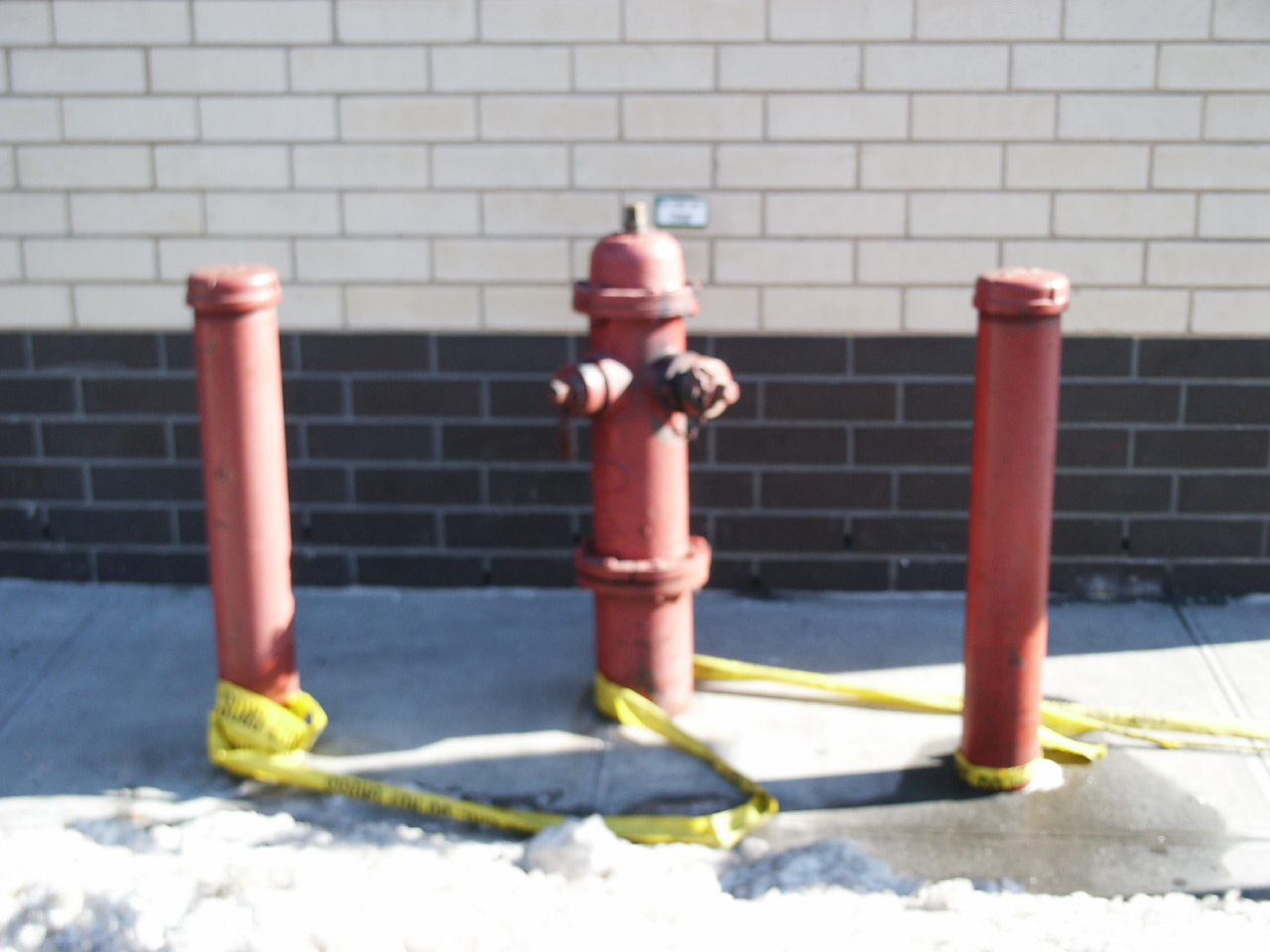In this slightly blurry color photo, a red fire hydrant stands centered on a concrete sidewalk, flanked by two red poles. The hydrant reaches up to waist height and has the necessary attachment points for fire hoses. Both poles, capped at the top, resemble sections of fire hydrants without the hose fittings. Yellow police tape is wrapped around the base of the leftmost pole and then twirls around the hydrant and the right pole, creating a snaking pattern. These elements are all positioned within two squares of the sidewalk, which appears wet and might be covered with snow. Behind the hydrant setup, a brick wall is visible, divided into two distinct sections: the bottom eight rows are dark brown or black, and the upper part consists of lighter cream or white bricks. Additionally, there's a shadow cast on the left side of the hydrant and poles, likely from a building.